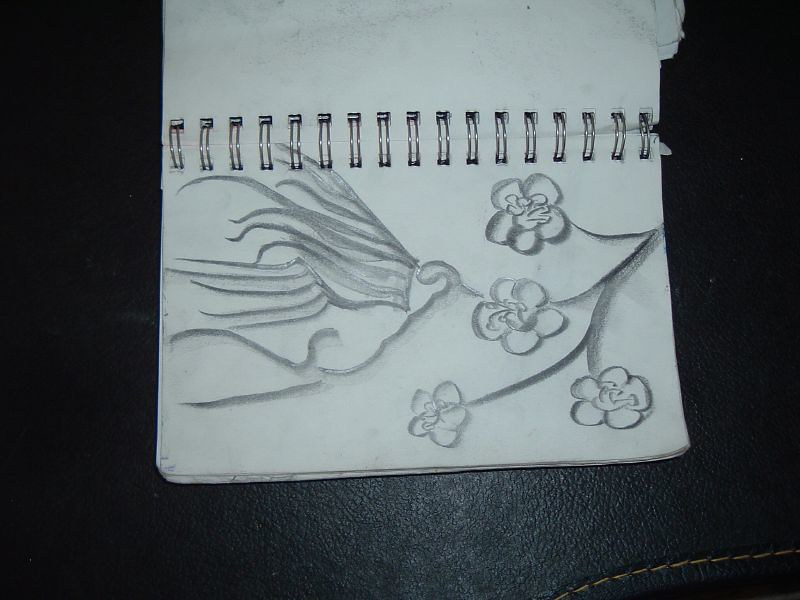This detailed photograph captures an open spiral-bound notebook laying on a black leather surface with tan stitching along the trim. The white pages, positioned horizontally, are opened to the middle of the book, revealing a hand-drawn pencil sketch. The drawing features a central motif of a branch with four flowers, where each flower has large rounded petals emanating from the branch. On the right side of the notebook, the flowers are arranged with one at the top, one in the middle, and two at the bottom. Slightly further left, the illustration transitions into wavy lines that could represent either hills or water. Above these lines, a delicate form resembling either a flying fish or a kite with long wispy protrusions is visible, creating a sense of motion. The page also has watermarks and pieces of paper sticking out, adding a textured visual interest.